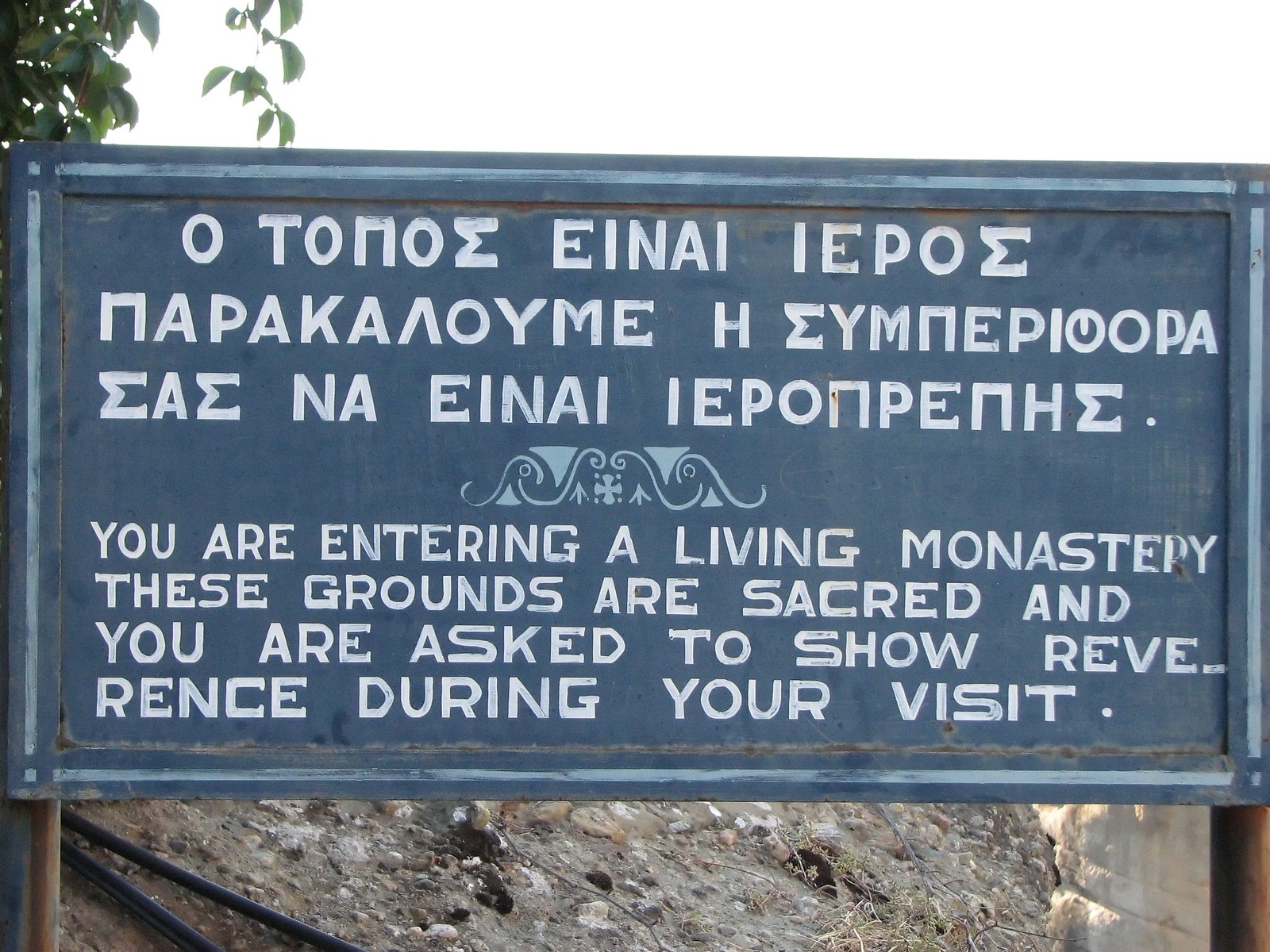In this outdoor setting, a large rectangular blue sign is prominently displayed against a backdrop of a rocky cliff and dirt ground, with tree branches hanging down on the left side. The sign is supported by metal posts that have a rustic, possibly wooden appearance. The sign itself, in a grayish-blue hue, features white capital letters. The top half of the sign is inscribed with Greek writing, and beneath this text, there is an abstract graphic that separates the Greek from the English translation below. The English translation reads: "You are entering a living monastery. These grounds are sacred and you are asked to show reverence during your visit." This sign serves as a respectful warning to visitors of the sacred nature of the monastery grounds.